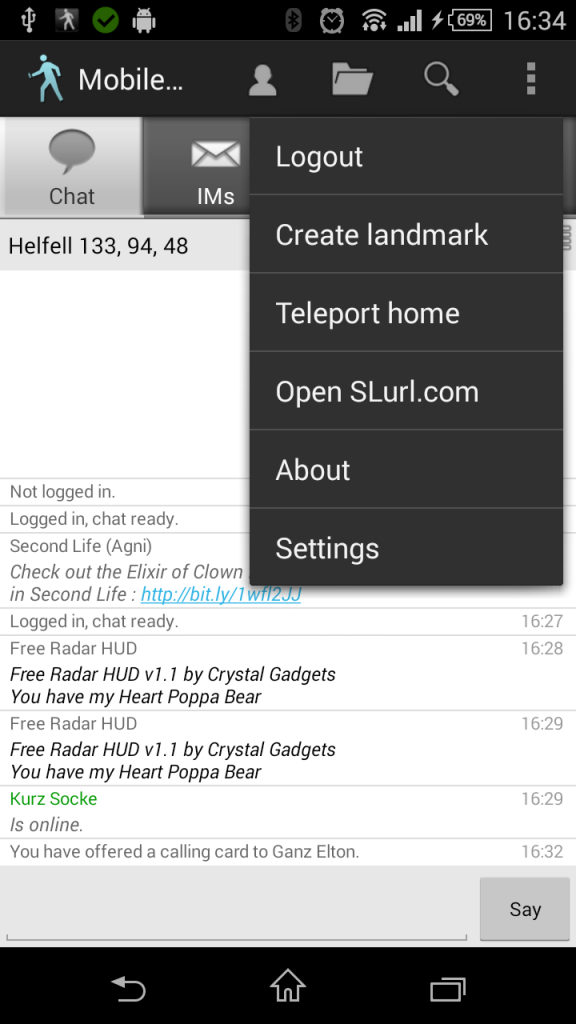The image is a screenshot captured in portrait mode, resembling a smartphone interface. In the upper left and upper right corners, there are various icons and elements typical of a phone display. On the upper right, a green circle with a check mark is visible, possibly indicating a notification or confirmation, next to an Android icon. Moving to the right, there's a battery icon showing 69% charge, and the time displayed as 16:34, all set against a black background.

Below this, the background shifts to a slightly lighter shade of black. A blue icon of a person walking leftward is visible, labeled "mobile." Alongside, there's an array of icons: a person icon, a folder icon, a search icon, and three dots indicative of additional menu options. An active menu is seen, featuring six options: "Log out," "Create landmark," "Teleport home," "Open slurl.com," "About," and "Settings."

Further down, another row starts with "Chat IMS," followed by what seems to be coordinates "Hellfell 133, 94, 48." Next is a large white space, likely a textbox or placeholder, with two subsequent rows stating "Not logged in" and "Logged in chat record ready." Another line reads, "Second life AG and I check out the elixir of clown in second light," accompanied by a hyperlink. Below, it says "Logged in chat ready" and "Free radar HRD HUD by crystal gadgets." There’s also the phrase "You have my heart Papa bear" which repeats.

At the bottom in green text, "KURZSOCKE is online" is prominently displayed. This comprehensive description captures all the visual details as well as textual elements found in the screenshot.